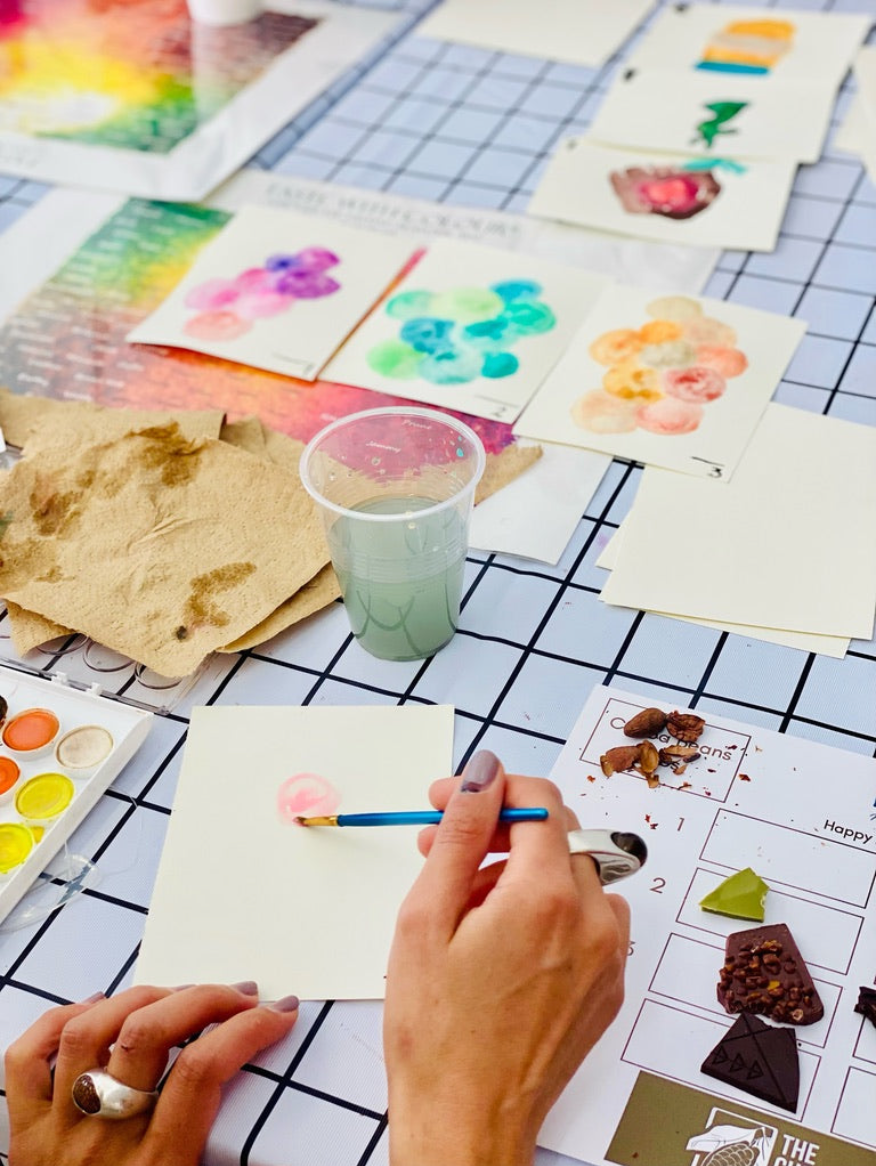In this detailed image captured indoors, a woman is immersed in her art, handling a blue paintbrush with her right hand while her left hand, adorned with a prominent silver ring, steadies a small rectangular piece of paper. She is meticulously painting a pink circle on the white paper. Surrounding her on the table, which features a light blue-gray surface with black grid-like lines, are numerous other small sheets, some filled with colorful watercolor paintings of clustered circles in hues of purple, pink, blue, green, orange, and beige, while others remain blank.

The table is cluttered with art supplies: a cup of greenish-brown water for rinsing the paintbrush, various containers of watercolor paints including shades of yellow, white, and orange, brown paper towels, and what seems to be a few broken snack pieces or cookies. On her left, traditional paint containers are visible, and to her right, there are materials seemingly used for making natural paints, such as cocoa beans and pieces of chocolate. Despite the busy scene, the focus of the image is sharply on her hands and the delicate act of painting, with the myriad of completed artworks creating a vibrant yet blurred backdrop.